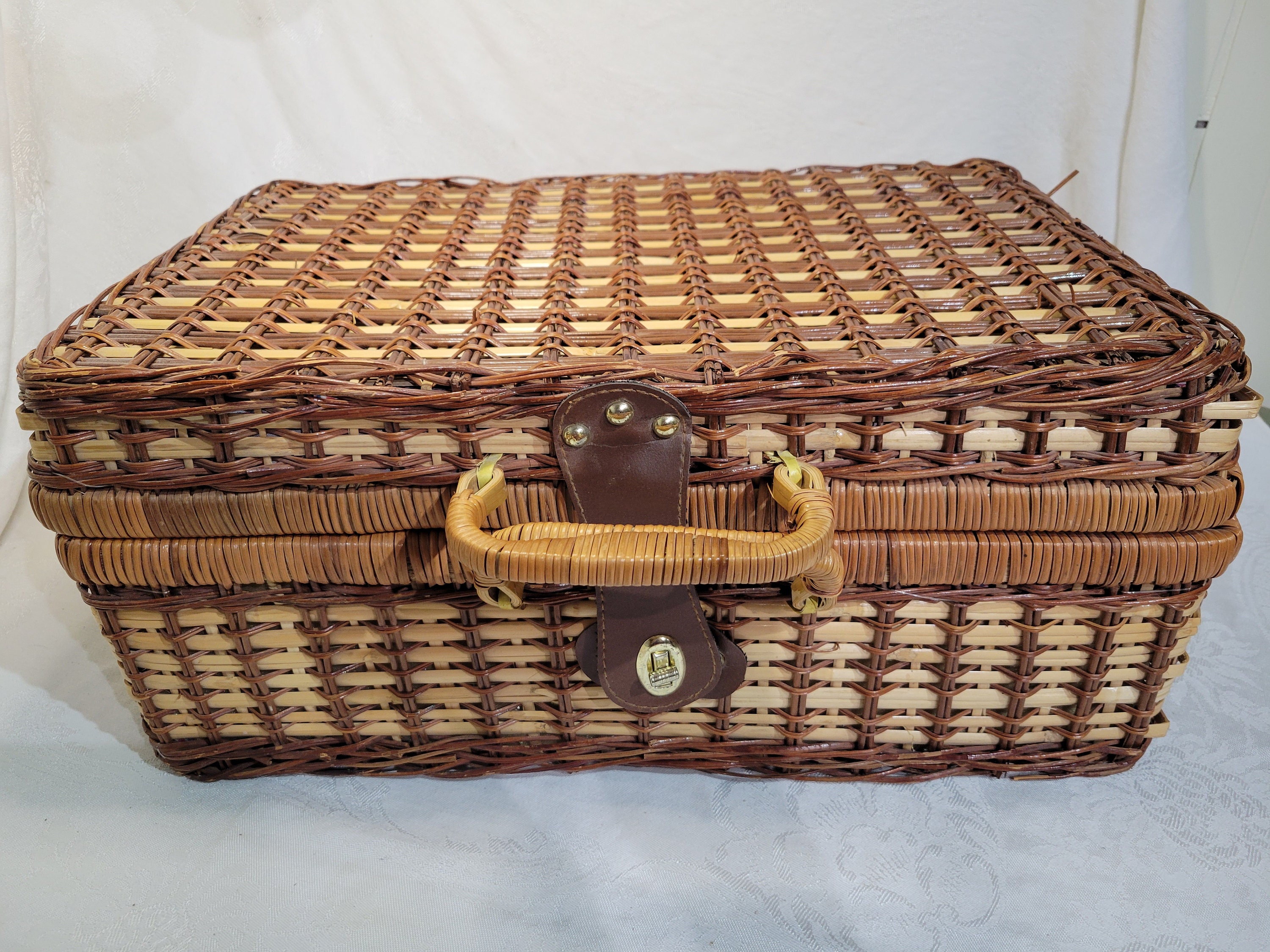The image captures an old-fashioned wicker picnic basket, designed like a suitcase, set against a white backdrop that looks to be part of a photo studio setup. The basket is constructed from a woven wicker pattern in shades of tan, brown, and orange, with darker colored wicker forming a grid or striped appearance. It features a pair of sturdy handles that are similar to those found on teapots, wrapped in a reed-type cord, and lay side by side. The basket is secured with a leather-like strap that clasps shut, adorned with three gold bolts and a crest-like logo, though the materials seem somewhat pleathery and newer, suggesting it might be a reproduction meant to look vintage. The wicker shows some wear and tear, with stray pieces visible. The basket, approximately two feet wide and one foot deep, is well-illuminated, highlighting its detailed craftsmanship and giving an impression of a carefully staged vintage artifact.